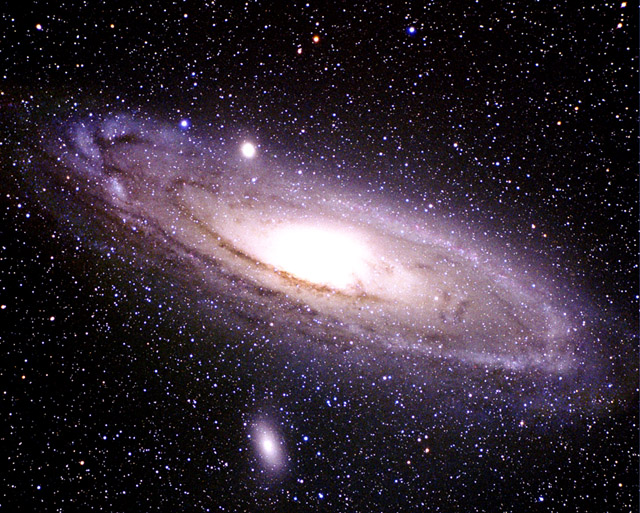This image captures a mesmerizing section of the Milky Way galaxy, set against a deep midnight blue or black background brimming with a multitude of stars in various colors, including blue, white, red, pink, and yellow. Dominating the center is a bright, almost blindingly white spherical object, reminiscent of a shining ball or possibly Saturn due to the notable rings encircling it. These rings create a swirling motion that gives an appearance akin to a hurricane or cloud-like formation. The swirl itself is illuminated in hues of purple, light purple, and magenta, adding a celestial glow to the overall composition. Surrounding the main object are several smaller bright points that could represent planets, stars, or even meteoroids, contributing to the intricate tapestry of the galaxy.